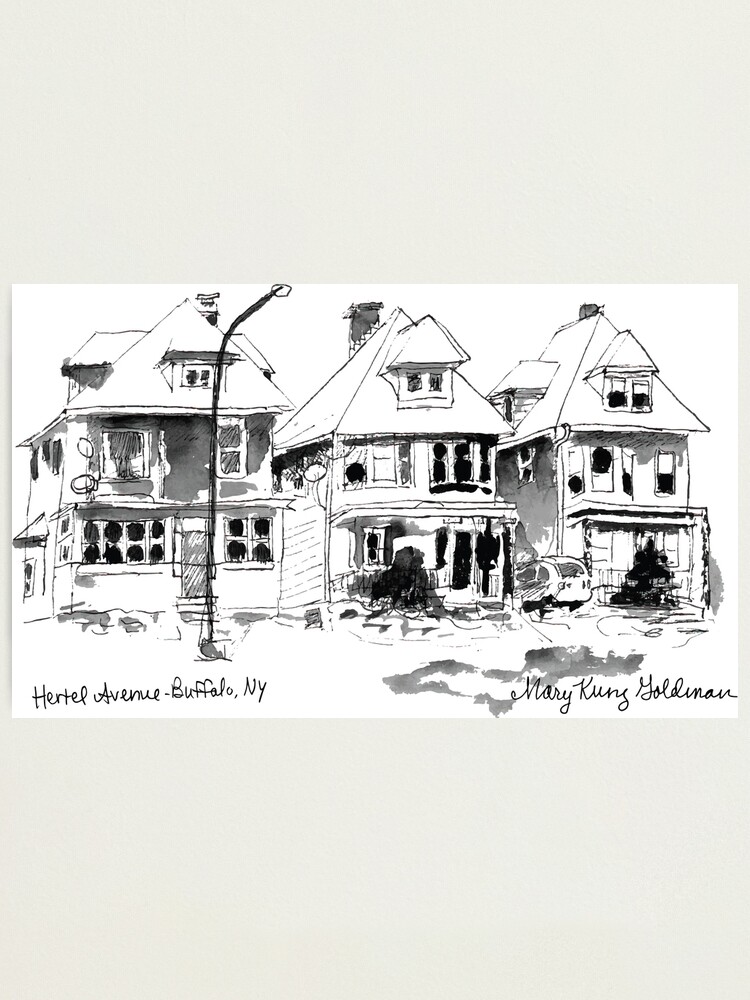This detailed black and white sketch depicts three closely situated, two-story houses reminiscent of 1930s and 40s summer homes near the Jersey Shore. These tall, narrow townhouses feature multiple windows, with some incorporating distinctive architectural elements such as gable pieces and bay windows. The house on the left boasts a closed-in porch framed by windows, possibly with snow hinted on its roof. The middle house, of a similar design, includes a prominent bay window on the top floor and has an open porch encircled by a railing. The house on the right, mirroring the others, shows a car parked in its driveway and a large bush in the front garden. All homes have triangular roofs with additional triangular dormer windows. The entire scene is captured meticulously in black and white, complemented by a detailed streetlamp on the left and grass indicated by squiggly lines. In the lower left corner, the sketch is labeled "Hertel Avenue, Buffalo, New York," and signed "Mary Kung Goldman" in cursive on the right.